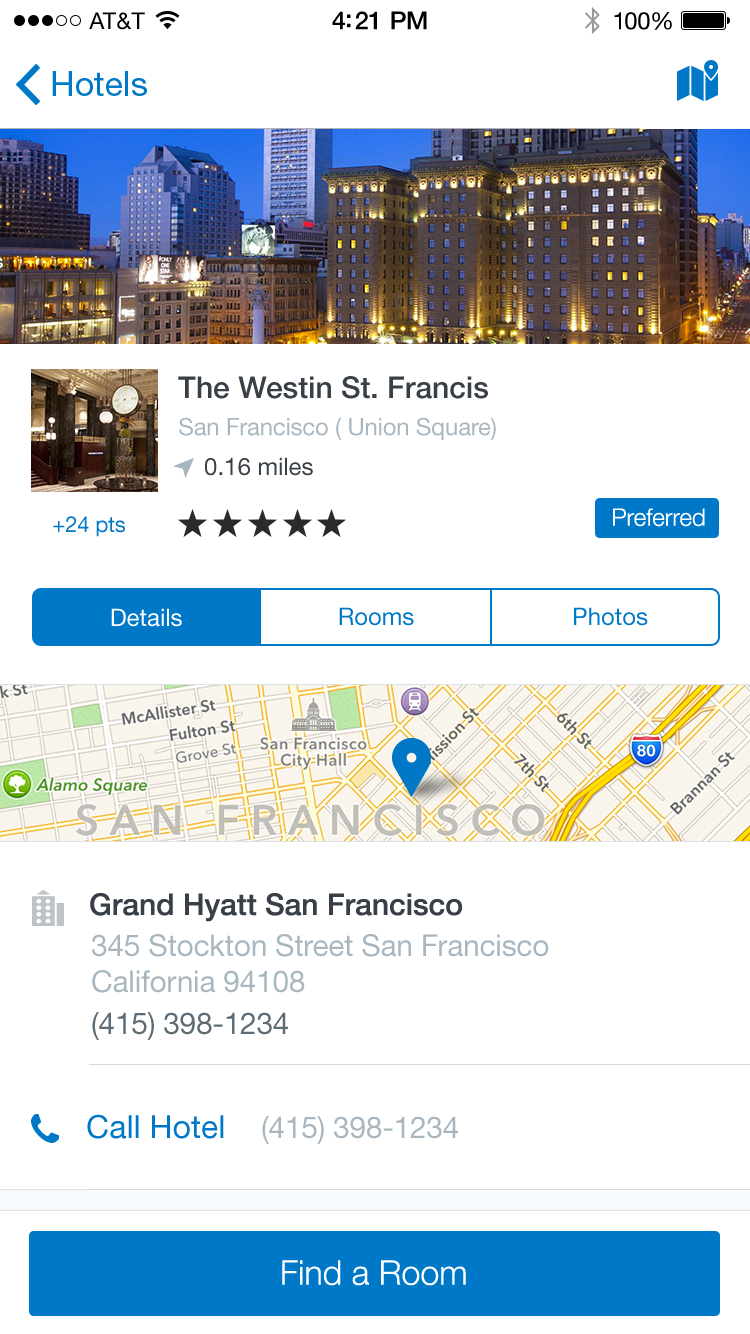The smartphone screen displays an AT&T network at the top, featuring Wi-Fi and Bluetooth icons along with the current time. Below the top bar, there's a blue back button labeled "Hotels," accompanied by a blue map icon.

The central part of the screen showcases an image of a cityscape with a prominent hotel building. It details "The Westin St. Francis, San Francisco, Union Square," located 0.16 miles away with a 5-star rating and offering "+24 points." Adjacent to this, there is a blue "Preferred" button. Tabs labeled "Details," "Rooms," and "Photos" are also present for further exploration.

A map section highlights San Francisco, displaying landmarks such as Alamo Square and San Francisco City Hall, with streets and highways clearly marked. Below this, detailed information for "Grand Hyatt, San Francisco" is provided, including the address "345 Stockton St., San Francisco, CA, 94108" and the phone number "415-398-1234." A "Call Hotel" button replicates the phone number.

The bottom of the screen offers a blue "Find a Room" button. The page predominantly features black text against a white background, punctuated by various maps and interactive buttons.